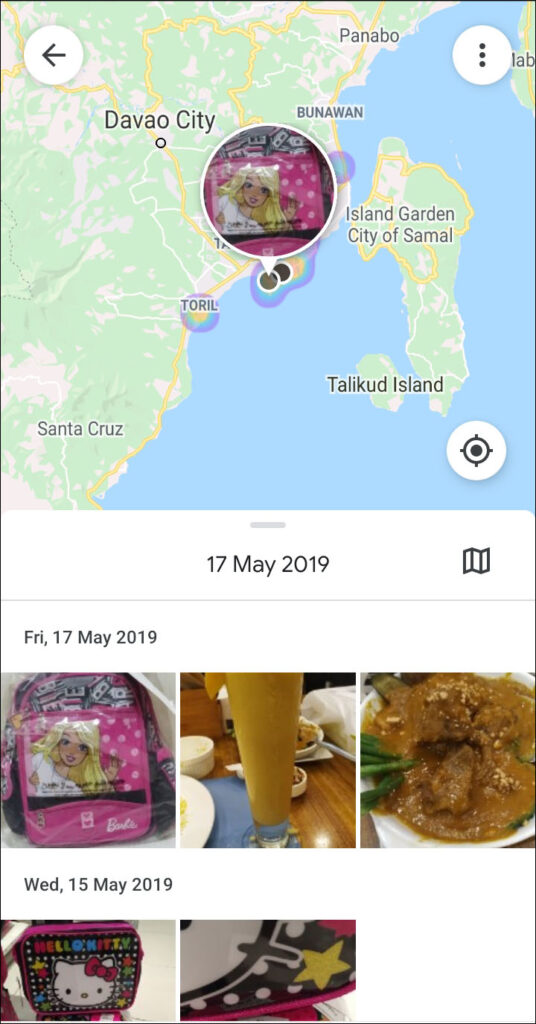The image is designed in a rectangular layout with a white background and a black border. It is divided into five sections, each containing different elements and images, arranged from the bottom to the top. Each section features a detailed visual clue or object of interest, marked with dates to indicate specific days.

The first section, at the very bottom, showcases a picture of a pink, white, and black Barbie book bed adorned with an image of a blonde-haired Barbie. This picture is accompanied by the text “FRI, 17th May 2009” written in black under a thin gray line. 

Moving upwards, the next section features a wooden table with a drink placed on it. The drink appears to be orange in color, and there are cut-off bowls also visible on the table. 

The third section displays a type of food that isn’t easily identifiable but includes what looks like green beans and another dish with green and brown hues. This section is followed by a white space with the text “WED, 15th May 2009” in black.

Above that, a close-up image of a Hello Kitty backpack is presented. The backpack features the iconic Hello Kitty face with a red bow and is surrounded by colors like white, black, orange, red, yellow, blue, and pink.

At the very top, the final section showcases a map predominantly in green, showing parts of water and marked locations such as Santa Cruz and Davao City. Overlaid on this map, there is an image of the Barbie picture from the first section, now presented in a circular frame with a pinpoint marking its location.

This arrangement provides a temporal and thematic narrative, guiding the viewer through different objects and contexts associated with specific dates.